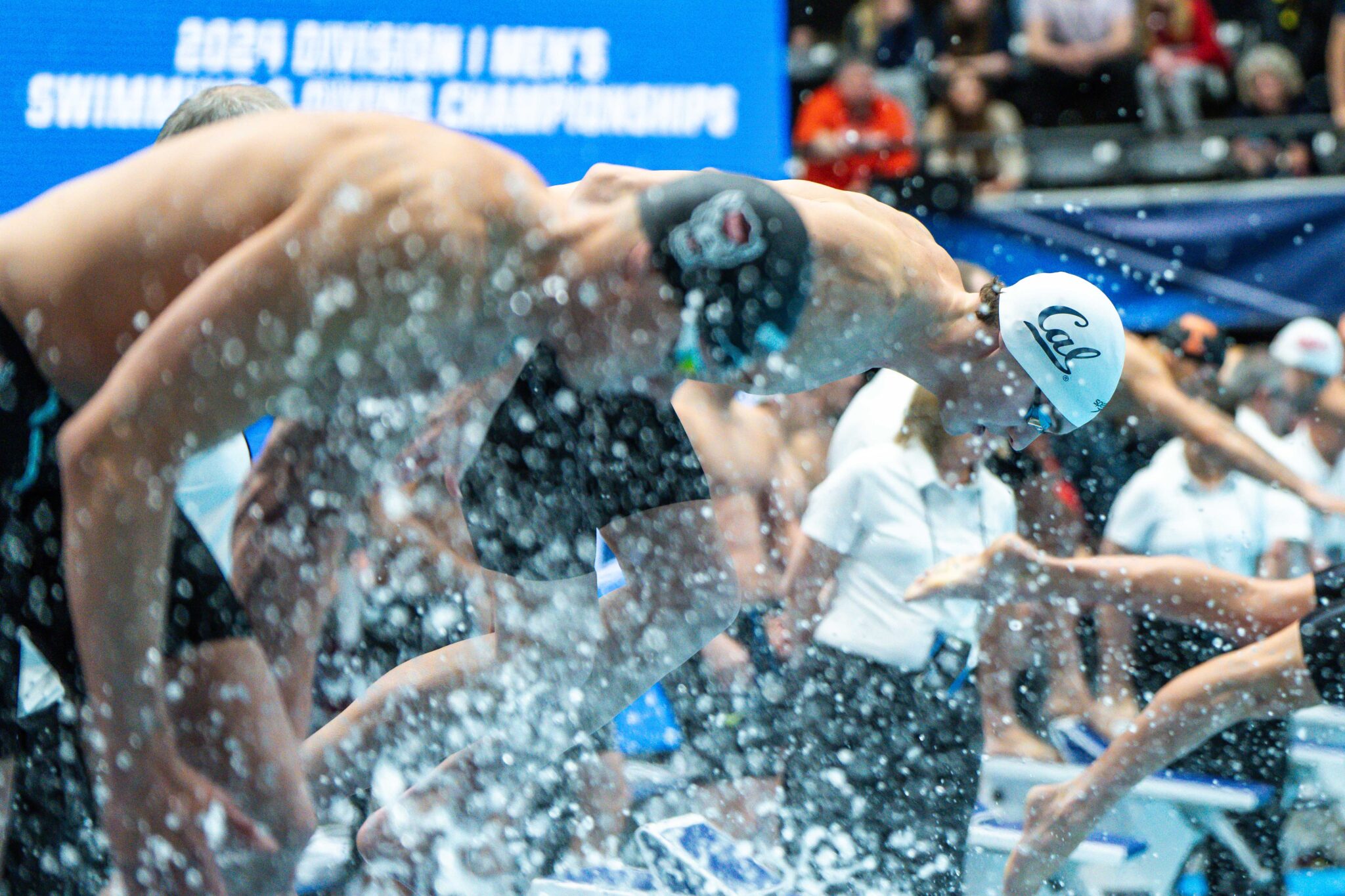The image captures the dramatic start of a race at the 2024 Division 1 Men's Swimming National Championships. In the foreground, three male divers are captured mid-dive, causing a splash of water that blurs parts of the scene. The closest diver, wearing black shorts and a black swim cap with goggles, is followed by another diver in black shorts with a white swim cap marked "CAL" in blue letters. Behind them, a third diver splashes into the water, distinguished by a University of Tennessee cap. The pool area is lively with various individuals, including judges near the diving platforms and spectators in the background dressed in an array of colors. A blue sign with white lettering, indicating the championship event, can be partially seen in the background, along with other indistinct figures and elements due to the motion and splash. The overall setting exudes the high energy and anticipation of a national competitive swimming event.